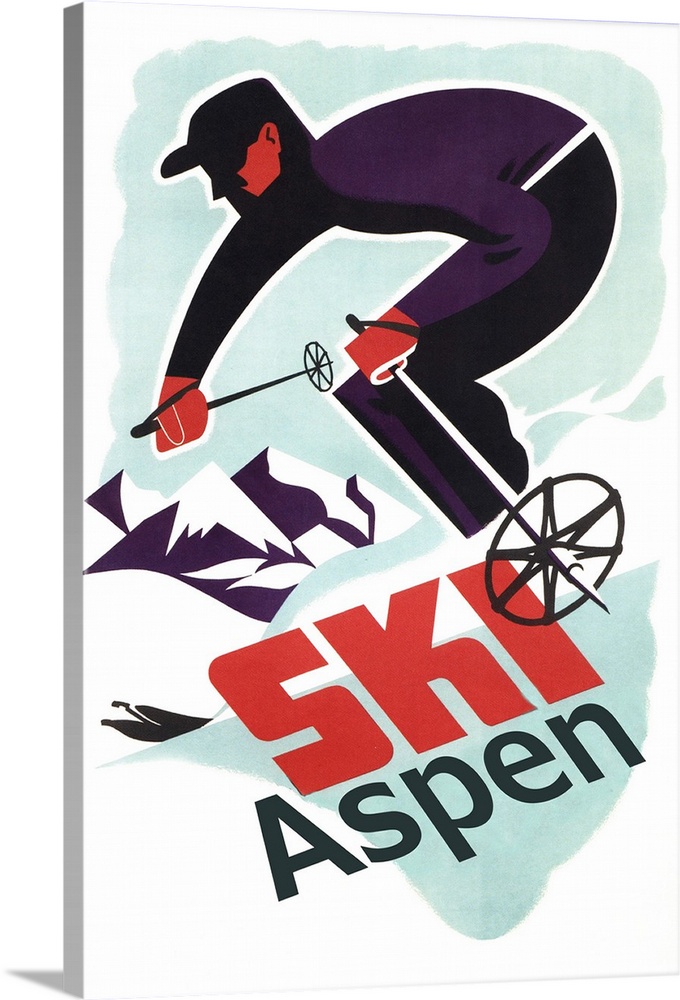This image appears to be a vintage-inspired travel poster for skiing in Aspen, rendered in a bold graphic style. Dominating the composition is the figure of a man in a skiing position, wearing a purple baseball cap, a dark purple long-sleeve shirt, and black and purple pants. His face is heavily shadowed, but the portion that's visible is red, matching the red of his mittens and the bold, blocky red letters spelling out "SKI" diagonally across the canvas. Below this, in smaller, minimal sans serif dark gray letters, is the word "Aspen." The man's ski poles are prominently superimposed over the text. The background features snow-capped mountains depicted in purple and white, with a mint green sky completing the scene. This detailed and eye-catching artwork is designed to promote Aspen as a premier skiing destination.